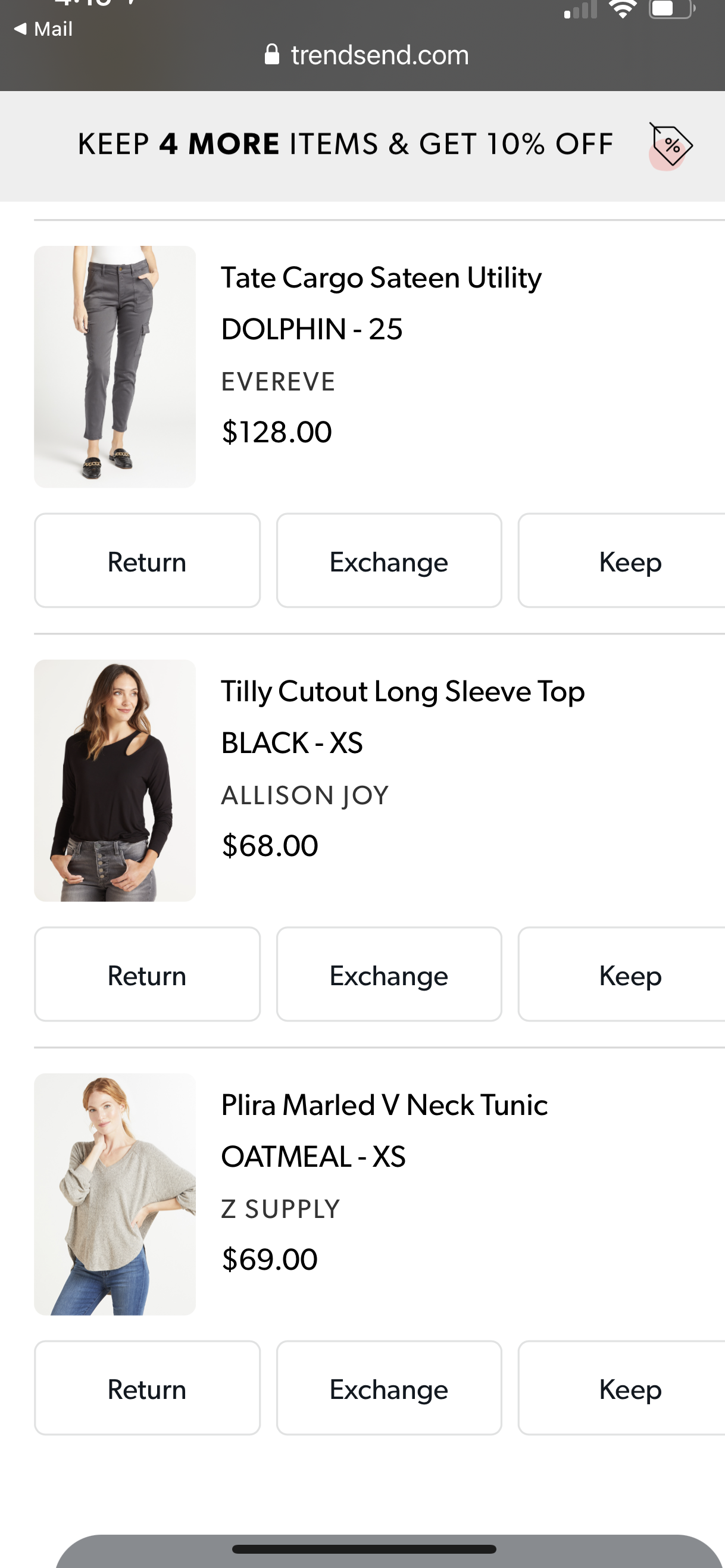The image appears to be a screenshot from a mobile device, likely a tablet, given its tall aspect ratio. At the top of the screen, there is a black bar displaying the URL "Trendsend.com," confirming the context of an e-commerce platform. Further reinforcing the mobile device assumption, the upper right corner features icons for battery life, Wi-Fi connectivity, and other wireless symbols.

Just below the black bar, there is a promotional banner that reads, "Keep 4 More Items and Get 10% Off," enticing the user with a discount offer. The main content area showcases three product listings, each accompanied by a picture of a woman modeling the respective apparel item. Each listing includes the item name, description, price, and three action buttons labeled "Return," "Exchange," and "Keep."

1. The first product is labeled "Cargo Satine Utility Dolphin-25 EVIR" priced at $128. The model is depicted wearing gray pants.
2. The second product is identified as "Tilly Cutout Long Sleeve Top Black-XS Allison Joy" with a price of $68. The model here is seen in a black shirt.
3. The third product is described as "Pira Marleed V-Neck Tunic Oatmeal-XS Z Supply," priced at $69, with the model wearing a gray shirt paired with blue jeans.

All three models appearing in the images are white women showcasing the diverse collection of trendy apparel offered by the site.